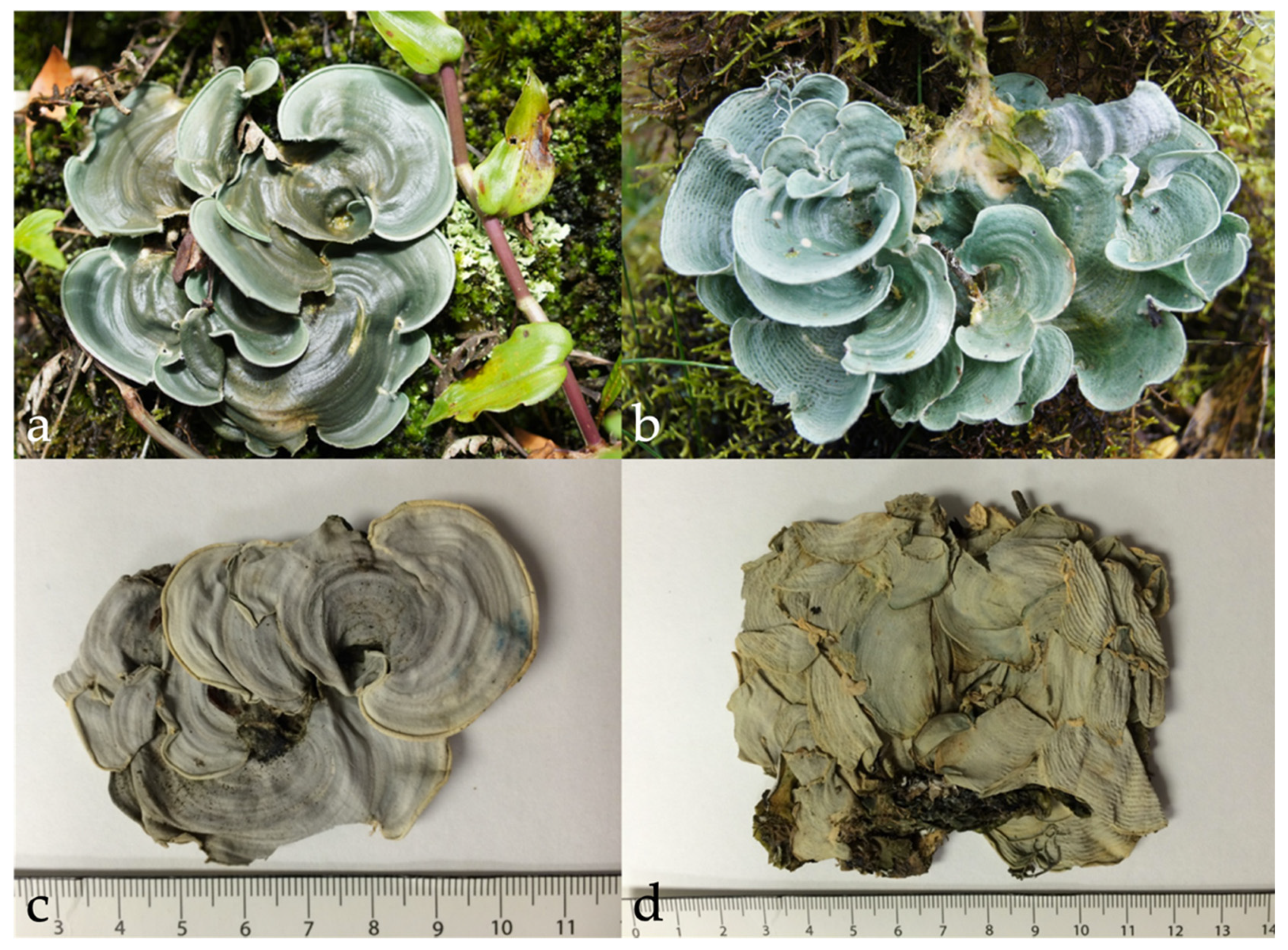The image is divided into four equal sections, labeled A, B, C, and D. Each section features photographs of plants or plant-like organisms at different stages. The images in the top row, A and B, display living specimens, while the bottom row, C and D, shows dried or decomposed versions of these subjects, measured with rulers.

- **Image A (upper left):** Features a living, light green lichen or moss growing outside, surrounded by greenery and seated on a bed of moss with some green leaves. It has a rounded, flowy appearance reminiscent of seashells crammed together.
  
- **Image B (upper right):** Another view of a living plant or lichen, this time more turquoise or light blue in color, and also surrounded by greenery. This specimen is also attached to brown sticks.
  
- **Image C (bottom left):** Shows the dried and flattened remains of the plant from Image A. The subject is dark gray, almost black, with a ruler beneath it indicating it measures 11 inches.
  
- **Image D (bottom right):** Displays the dried and flattened remains of the plant from Image B. This specimen has a greenish, pea-like color and also has a ruler beneath it showing it is 9 inches long.

The background colors for the dried specimens in Images C and D are gray and white, respectively, enhancing the contrast with their measured remains.